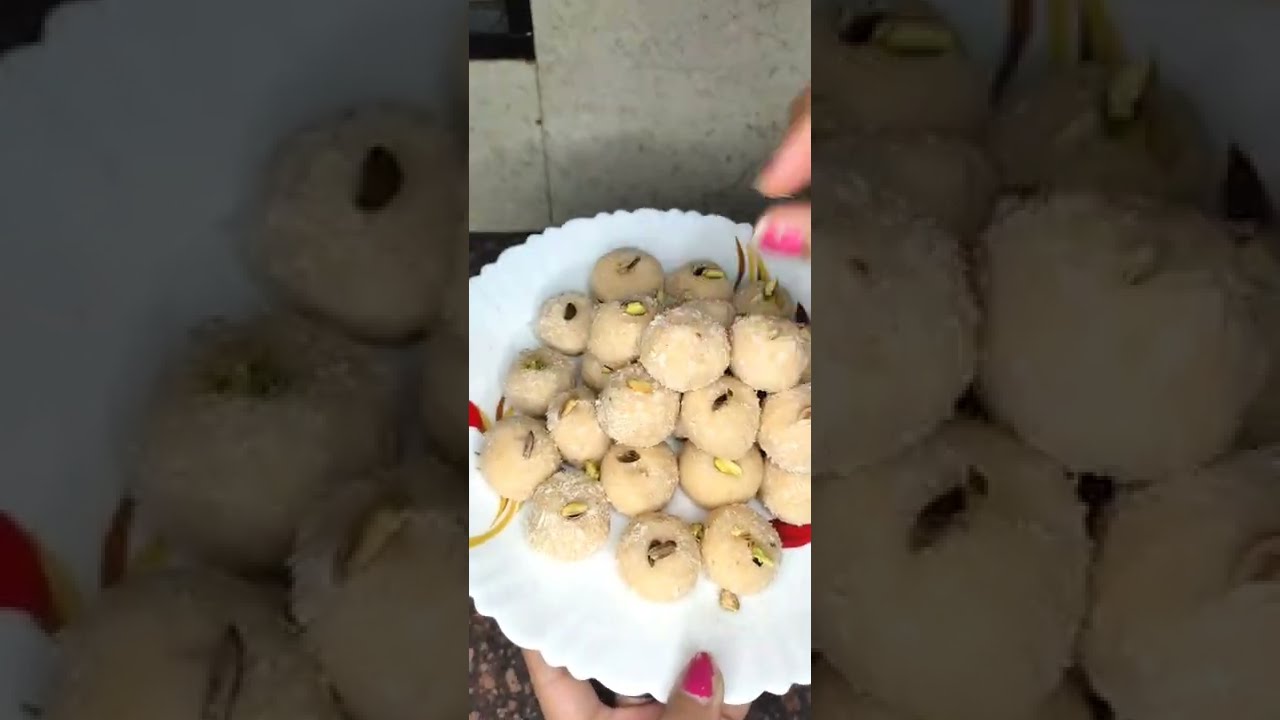The image depicts a close-up, personal photo of a white, scalloped-edge plate adorned with approximately 20 small, round cookies or dessert balls, each topped with what appears to be a pecan or a pistachio. The cookies, light tan in color, have a dusty or flaky appearance, as if coated in powdered sugar. The plate is held by a woman with light skin, showing fingers with chipped, pink nail polish. The composition is centered on the cookies, with two fingers and a thumb visible holding the plate. Additionally, elements of the same image appear to have been darkened, enlarged, and used as a background framing the central photo. Some faint hints of red and gold ribbons add to the festive feel of the scene.